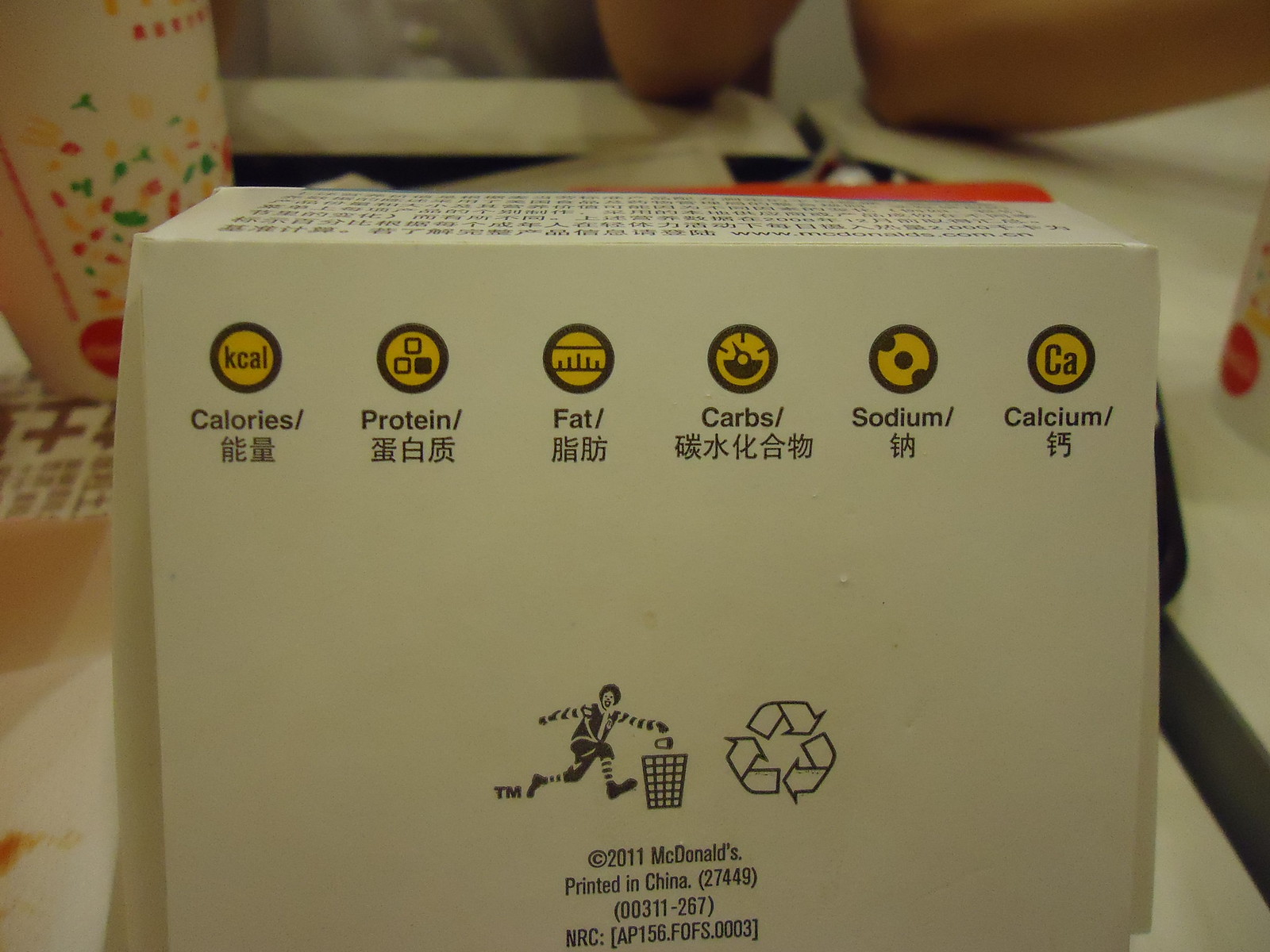In this photo, we see a McDonald's product packaging marked with "Copyright 2011, McDonald's" at the back. Prominently featured is an image of Ronald McDonald tossing litter into a wastebasket, emphasizing the importance of proper waste disposal. To the right of Ronald, there is a recycle symbol indicating the packaging's recyclability. Below this section, the text "Printed in China" is visible.

At the top of the packaging, from left to right, there are symbols representing calories, protein, fat, carbohydrates, sodium, and calcium. Each symbol is accompanied by its respective English word, and beneath these English terms, corresponding Chinese translations are printed. This bilingual approach ensures the information is accessible to both English and Chinese readers.

Additionally, the upper portion of the box is filled with Chinese characters, providing supplementary information in Chinese, further highlighting the product's target audience and manufacturing details. The detailed nutritional icons and bilingual text are a testament to McDonald's effort to cater to a diverse customer base while promoting environmental responsibility.